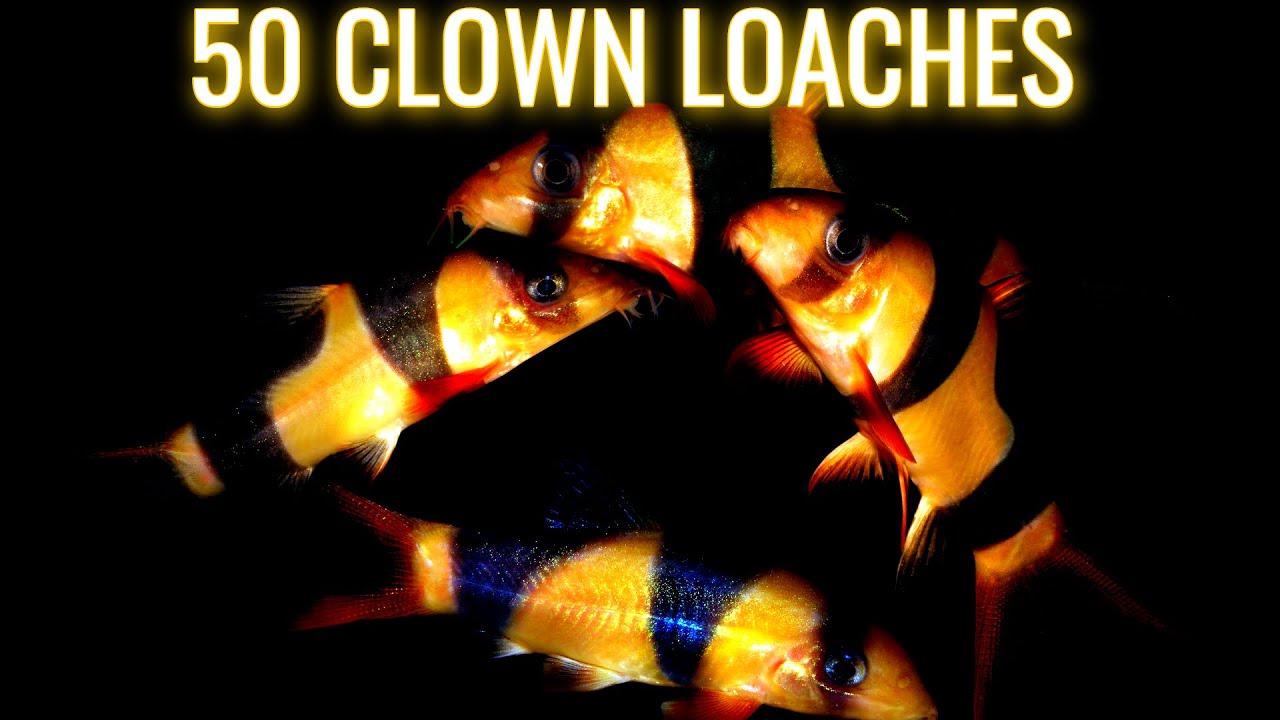In this striking image, set against a solid black background, four vibrant clown loaches are illuminated dramatically by a light. The fish, with their brilliant orange and gold bodies, are adorned with distinct dark stripes. Three of the fish feature black stripes while the fourth, situated at the bottom, boasts striking cobalt blue stripes. Their small black eyes are clearly visible, adding to their enchanting appearance. The fish appear to swim in a loosely circular formation. Above this captivating scene, well-lit white and yellow text reads "50 Clown Loaches," highlighting the name of these beautiful creatures.